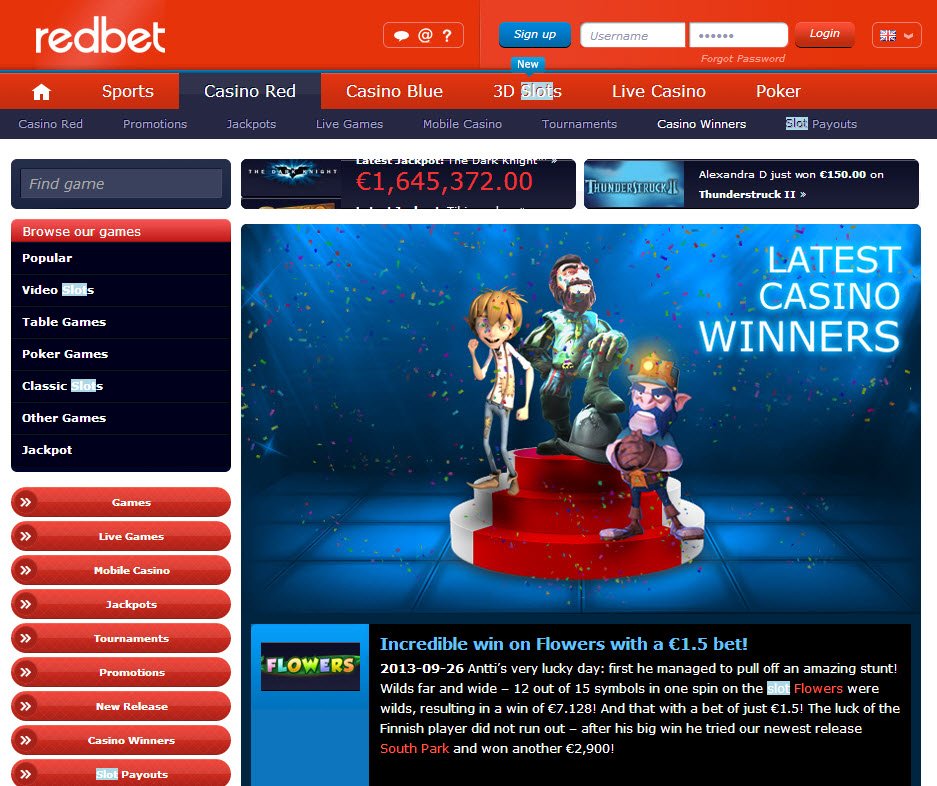This is a detailed screenshot of the Redbet website showcasing its navigation and core functionalities. The website's background is predominantly white, creating a clean and professional layout.

**Top Banner and Navigation Bar:**
- The top banner is a striking red, immediately catching attention.
- On the left-hand side, it features the site name "Redbet" in a unique font, likely serving as the logo.
- Towards the right of this banner, there's a small box with three white symbols: a chat symbol, an "@" symbol, and a question mark symbol.
- Adjacent to this box is a blue button labeled "Sign Up" in white text.
- There are two text boxes for entering a username and password, followed by a red "Login" button in white text.
- To the far right corner, there's a language drop-down box displaying the Union Jack, indicating the site is currently set to English.
- Below the password text box, in small white font, it states "Forgot Password?"

**Secondary Navigation Bar:**
- A thinner red bar below the top banner contains navigation buttons. These include icons and labels for: 
  - Home (house symbol)
  - Sports
  - Casino Red
  - Casino Blue
  - 3D Slots
  - Live Casino
  - Poker
- "Casino Red" is highlighted in black, showing it is the active tab.
- Further sub-options under this tab include: Casino Red, Promotions, Jackpots, Live Games, Noble Casino, Tournaments, Casino Winners, and Slot Payouts.

**Main Content:**
- The main body of the website has a white background with the primary focus on three rectangular segments at the top. 
  - The first segment is a dark grey search bar labeled "Find Game."
  - This is followed by banner ads; the first with a symbol that resembles Batman next to a euro total (1,645,322 euros).
  - The second banner advertises "Thunderstruck" with a light blue background, mentioning "Alexandra D just won 150 euros on Thunderstruck."

**Left Column:**
- The left-hand side of the site features red buttons for navigation:
  - The first button says "Browse Our Games" in white text.
  - Against a black background, other categories are listed: Popular Video, Table Games, Poker Games, Classic Slots, Other Games, and Jackpots.
  - Below these options are nine capsule-shaped buttons, each with a right-facing arrow.

**Main Display:**
- The central display is an image that appears to be a still from a game, bordered in black with a light blue background resembling an underwater scene.
- In the top right corner of this image, "Latest Casino Winners" is displayed, featuring details of an "incredible win on flowers with a 1 euro 50 bet." The image includes three characters standing on a three-layered circular platform, with additional information about the win provided below.

This comprehensively structured layout ensures clear navigation and highlights essential information effortlessly for users.